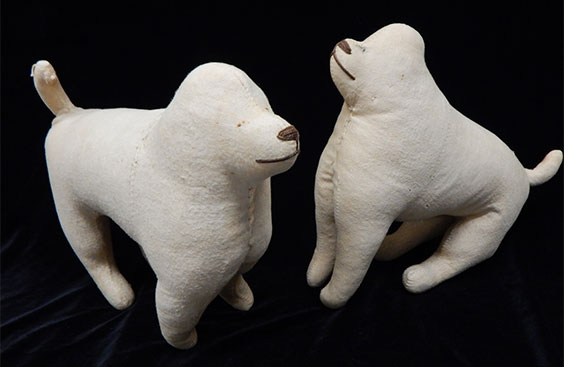The image depicts two simplistic, handmade clay dog figures posed against a black background. Both figures are crafted from a smooth, white material, giving them a sleek and minimalist appearance. The dogs are devoid of intricate details, sporting only basic outlines for their mouths, noses, and small, dot-like eyes. Notably, they lack any visible ears and fur, contributing to their streamlined look. One dog is standing on all four legs, facing left, while the other is sitting on its hind legs, looking upwards, perhaps towards an unseen owner. The latter is positioned on the right-hand side of the image. Each dog features a short, curved tail, and their heads are round and smooth. The overall impression is one of charming simplicity and understated craftsmanship.